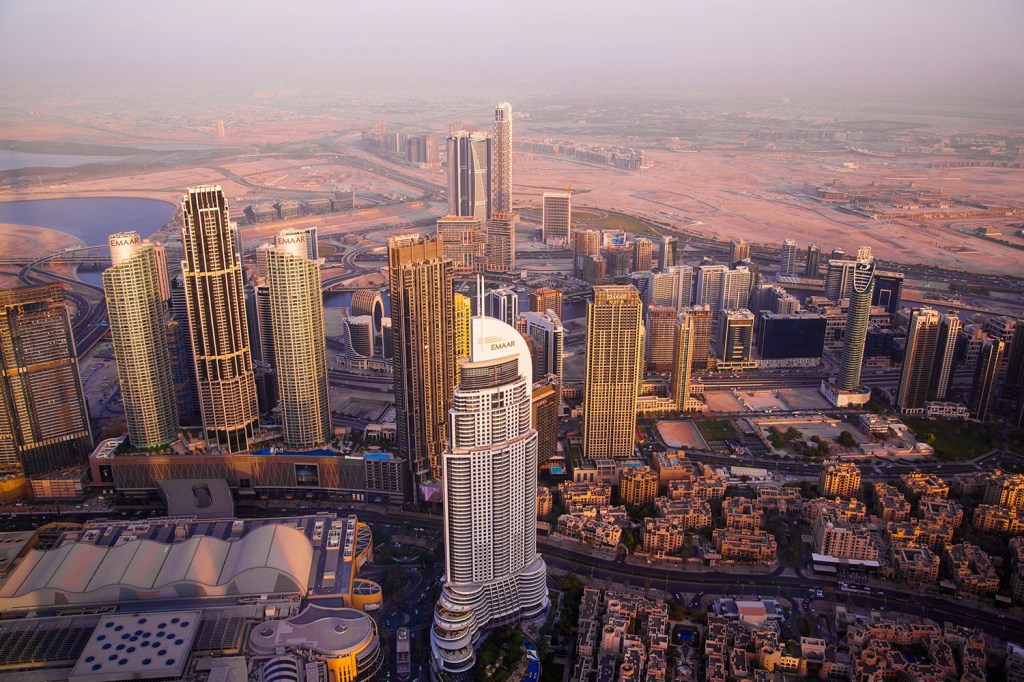An aerial, landscape-oriented color photograph offers a striking view of a bustling desert city. The cityscape features several closely-packed skyscrapers, particularly on the left where the tallest buildings tower over a mix of shorter ones. In the center stands a light gray building adorned with a distinctive white arched sail shape on its top, marked with the partially legible text "Dakar." Vehicles travel along a prominent road that cuts through the city's core, with another road lying behind the main cluster of buildings. On the left, a long bridge spans over a visible body of water. Additionally, the city includes an area with warehouse buildings characterized by Quonset hut-style roofs, specifically located in the left foreground. The scene lacks greenery, except for a few short trees in the right middle section, and the background transitions into a vast expanse of red and beige desert sand under a hazy gray sky.